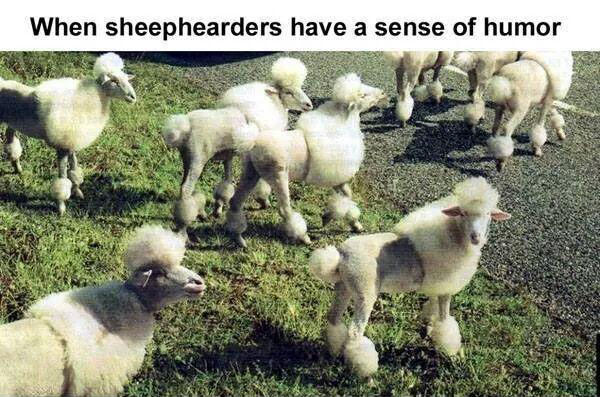The image features a group of approximately eight sheep, some partially out of frame, humorously groomed to resemble poodles. Their distinctive haircuts leave their upper bodies, heads, tails, and ankles fluffy, while their midsections are shaved. The sheep are split between standing on a green grassy area and a paved road marked with white lines, all seemingly poised to cross the street. At the top of the image, there is a caption in black text on a white background that reads, "When sheep herders have a sense of humor." The amusing contrast between the sheep's natural state and their novel haircuts provides a whimsical scene of sheep farming.